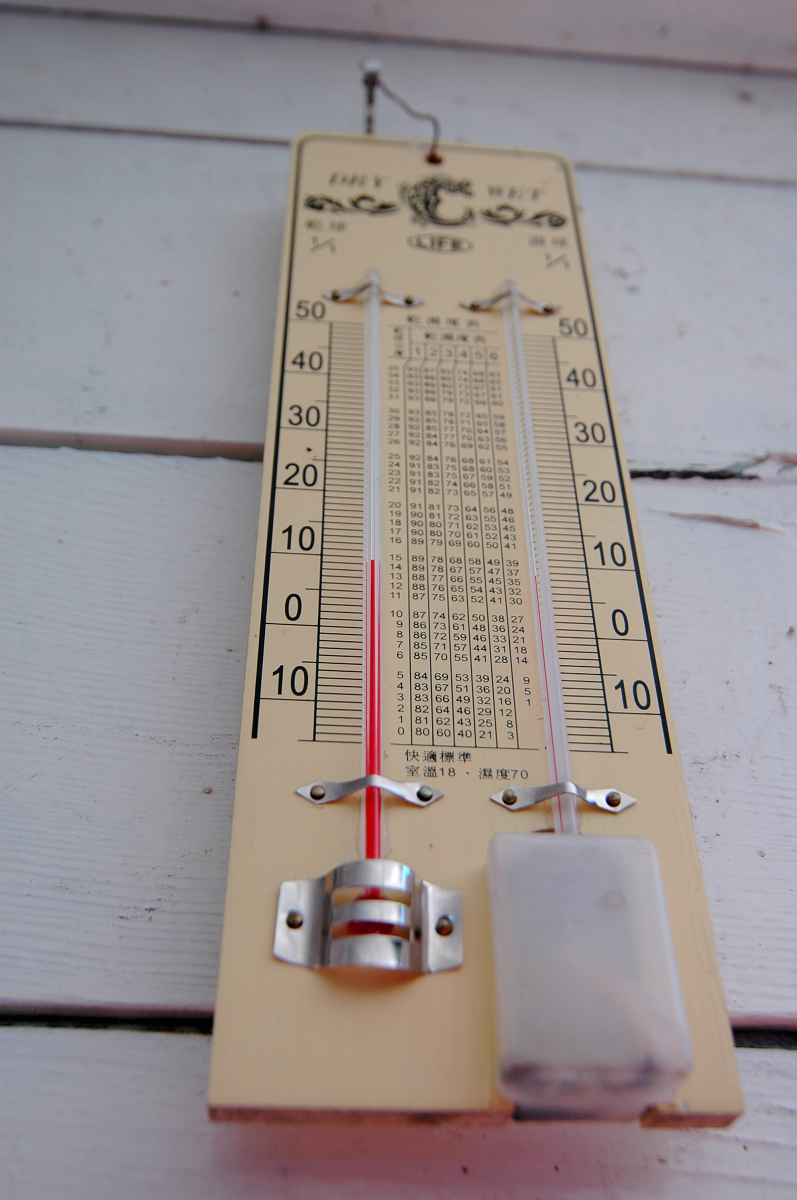This photograph features a wall-mounted thermometer viewed from a lower angle, which makes it difficult to determine its exact size. The thermometer appears to be installed on the exterior wall of a garden shed or similar structure, as indicated by the white-painted wooden horizontal slats in the background.

The thermometer itself consists of two vertical glass cylinders that display the temperature. Both cylinders contain visible red lines: the left cylinder features a thicker red line that reaches up to around the 10-degree mark, while the thinner red line in the right cylinder stops just below the 10-degree mark. 

The left and right sides of the thermometer are marked with large, identical numerical labels. These numbers increase in increments of 10, ranging from 0 at the bottom to 50 at the top. These larger numbers are accompanied by smaller vertical lines representing minor divisions between each set of larger numbers. Although not explicitly labeled, these lines provide more precise temperature readings.

The central area between the two thermometers contains a grid of numbers, though their exact purpose is not immediately clear. At the very top of the thermometer, some text is faintly visible but out of focus, rendering it unreadable. The overall scene hints at a well-organized garden or outdoor area, possibly maintained meticulously, given the condition and placement of the thermometer.